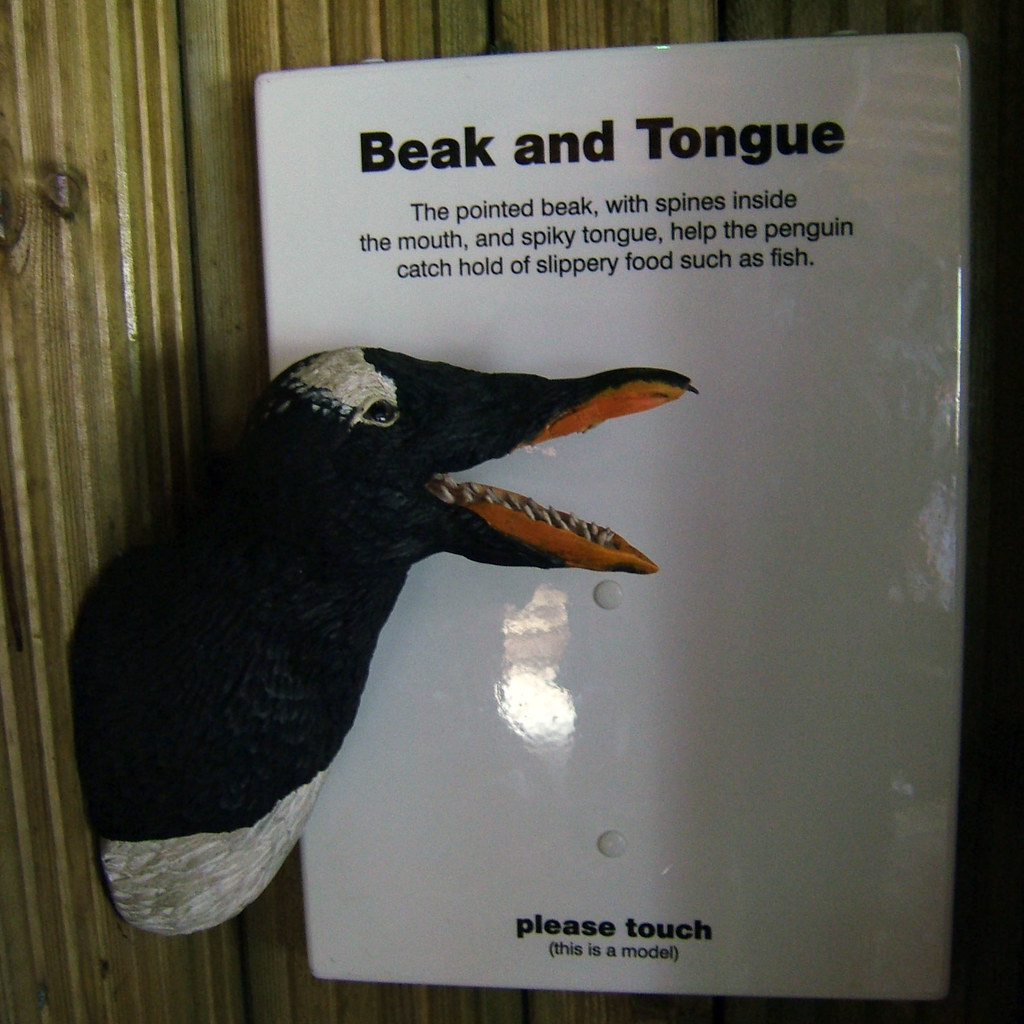In this image, set against a vertical bamboo-like wooden background, we see an indoor display that appears to be from a museum or zoo. The focus is on a mounted penguin head sculpture positioned near the center of the image, overlapping a white informational plaque to its right. The penguin sculpture features detailed elements such as a black head, a white eye, and a brown interior mouth showcasing spiked spines, all made to look realistic though handmade or taxidermy. The plaque, in dark black letters, bears the title "Beak and Tongue" at the top. Below this, it explains that the pointed beak and spiky tongue help penguins catch slippery food like fish. The sign concludes with an invitation to interact, stating "Please touch. This is a model." Various shades of brown, black, orange, white, and tan dominate the color palette of this detailed and educational exhibit.